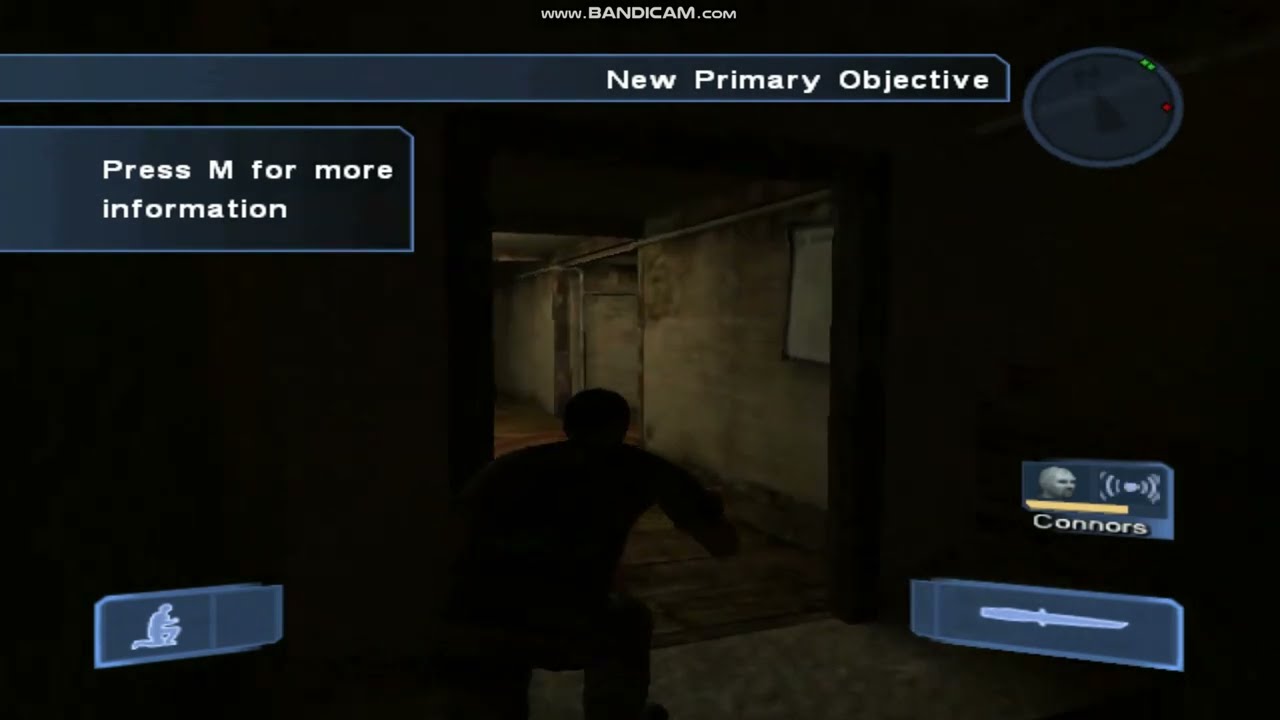The image is a horizontal screenshot from a video game, evidencing the website "www.bandicam.com" in small white letters at the top middle. The scene is dark, depicting the silhouette of a character who appears to be crouching, possibly indicating stealth gameplay like in a spy game. The character is poised to enter a poorly lit hallway with grimy walls and a dirty floor, transitioning from a concrete-floored area to one with wooden flooring and stone walls streaked with darker brown.

At the top of the screen, framed by a blue shaded border, is the text "New Primary Objective" in white letters. On the left side, another blue-bordered element reads "Press M for more information." On the lower right corner, the HUD includes the face of a character labeled "Connors" with a yellow bar beneath it. Below this, another bordered rectangular section, also shaded in blue, displays an image indicative of a weapon, likely a knife, suggesting that the character may be armed for melee combat. The overall dark setting and the stealthy, armed character hint at a game with espionage or survival elements.